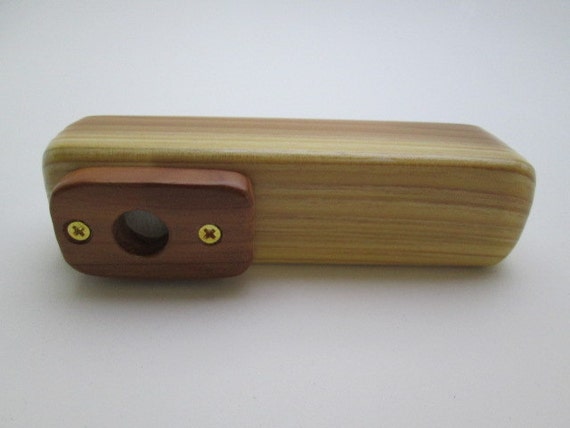This image is a high-resolution color photograph capturing a smoothly finished wooden piece. The wooden object, which seems to be either a square block with rounded edges or possibly a curved shape, is predominantly a light brown hue adorned with dark brown grain patterns. The object's backside is not visible, adding an element of intrigue about its overall form. Affixed to the top portion of the front-facing side is a small, flat rectangular attachment with elegantly curved edges. This attachment, fastened with gleaming gold screws, features a centrally located circular hole, suggesting a functional or decorative purpose. The attachment is made from wood of a medium brown shade, distinguished by its visible grain patterning. The expertly crafted assembly of these components hints at the object being a piece of artisanal woodwork, potentially a toy or another type of decorative wooden item.